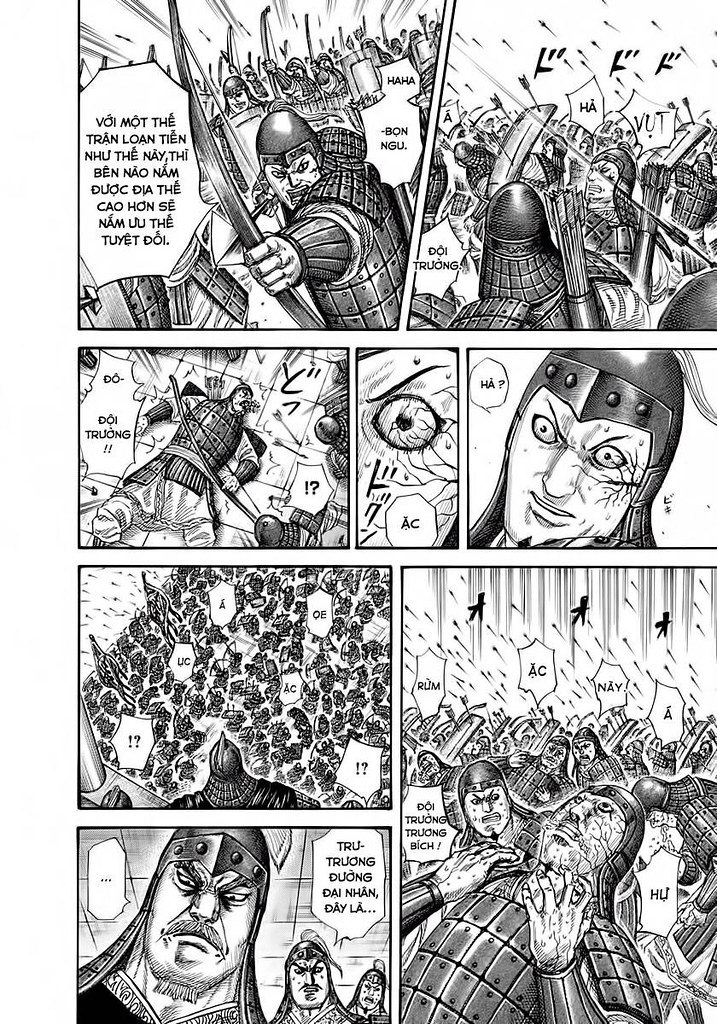The image is a detailed black-and-white scanned comic book page, presented in a window pane style format, making it easy to follow. The text within the panels is written in Vietnamese, with one of the words being “haha.” The scene primarily features a large group of soldiers, reminiscent of a Spartan army, equipped with diverse gear, shields, and armor. The artwork showcases dynamic scenes, including one where a person at the top of the page is preparing to shoot a bow and arrow, which then appears to hit an individual. Another striking detail is an eye with veins visibly popping out. The overall visual narrative suggests a setting filled with warriors, fighting sequences, and intense moments, indicative of a comic book that might originate from a different country or be part of a newspaper comic strip.